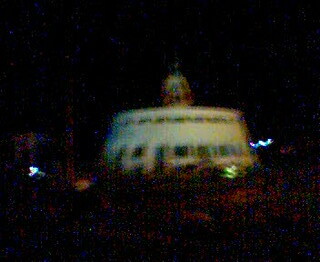A very blurry image captures a colorful round building shrouded in darkness. Despite the poor lighting, the structure's white exterior adorned with a myriad of vibrant hues stands out. The building features numerous windows, each framed with a spectrum of colors. At the rooftop, a rim decorated with small, colorful patterns encircles the building. Rising above this rim, a tower similarly painted white with vivid red accents pierces the night sky. On either side of the building, faintly visible blue light squiggles add a whimsical touch, in addition to a green squiggle towards the base. The surroundings of the building are obscured by the darkness, offering only a glimpse of the colorful architecture within a shadowy environment.